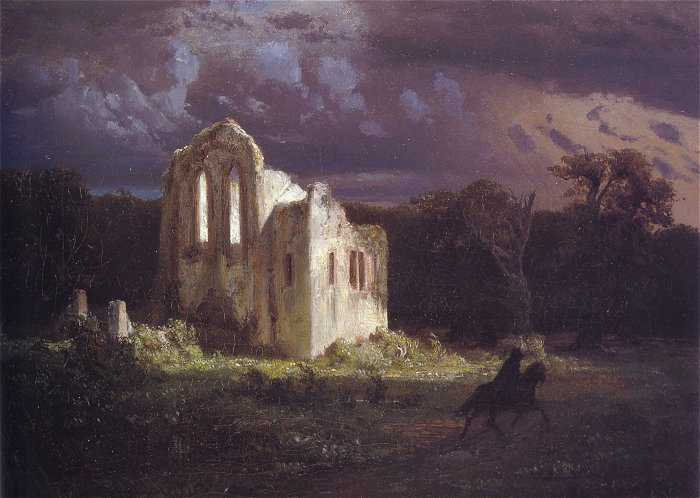The image is a detailed and atmospheric painting set in a dark, likely nighttime scene. The sky is dominated by deep, stormy hues of purple and blue, with wispy gray clouds that seem to be dissipating. On the ground, there's a mix of dark land and patches of green, indicating a field with grass, bushes, and wiry, leaning trees. The focal point on the right side of the painting is a shadowy figure of a person riding a black horse, both appearing as silhouettes against the darker background. Towards the left of the scene, there's a prominent, dilapidated white building, possibly the ruins of a castle or church. This structure looks ancient, with parts missing and signs of rust and overgrowth of vines and plants, contributing to its worn and mystical appearance. The sky's muted light appears to give the building an eerie illumination, though the light source is not clearly visible, adding to the painting's mysterious and haunting ambiance.